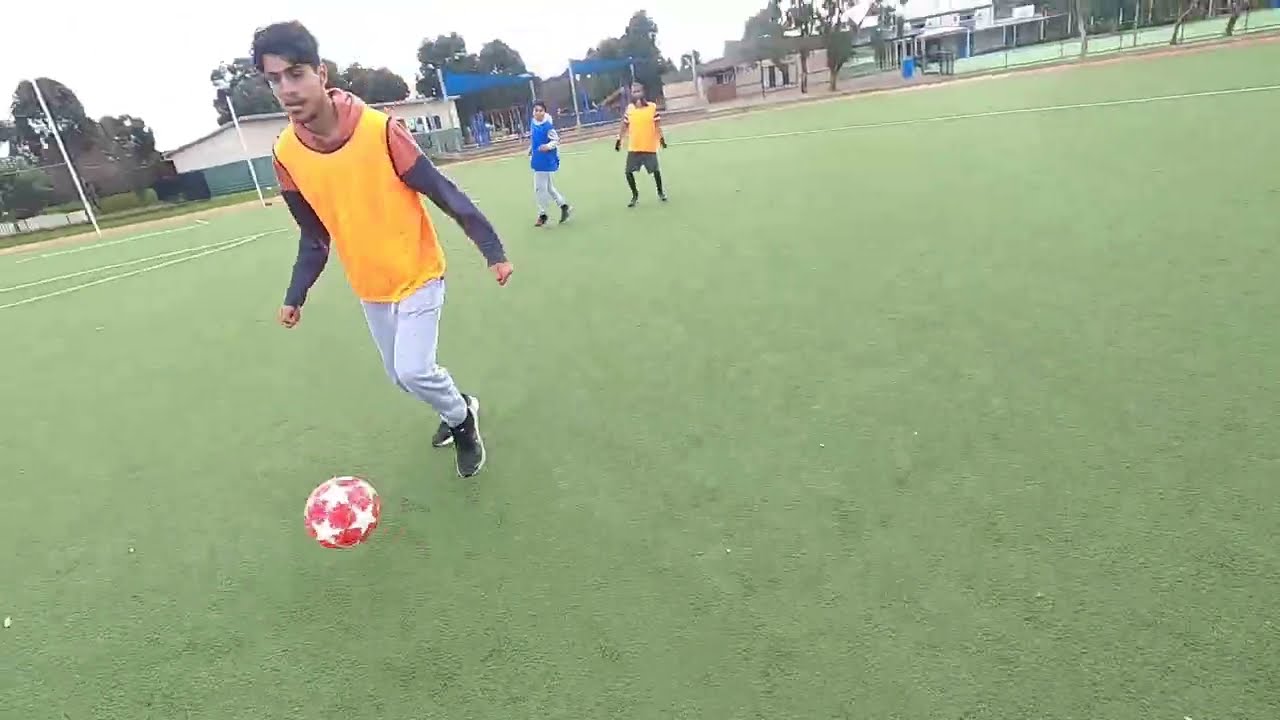The image captures a lively outdoor scene of boys playing soccer on a lush green turf field. Prominently featured on the left-hand side is a young Latino boy with brown skin and black hair, clad in a yellow pinnie over a hoodie, gray sweatpants, and black shoes. He is actively kicking a red soccer ball adorned with white stars. Behind him, two boys can be seen, one wearing a yellow pinnie and the other a blue one, indicating opposing teams. The backdrop includes a fence, a beige house, and a white building to the right. Additionally, white poles with a blue flag can be seen across the upper part of the image, suggesting a school or sports facility setting amidst green trees in the distance. The overall scene appears to capture the dynamic action of a soccer match, possibly during a school gym or PE class.